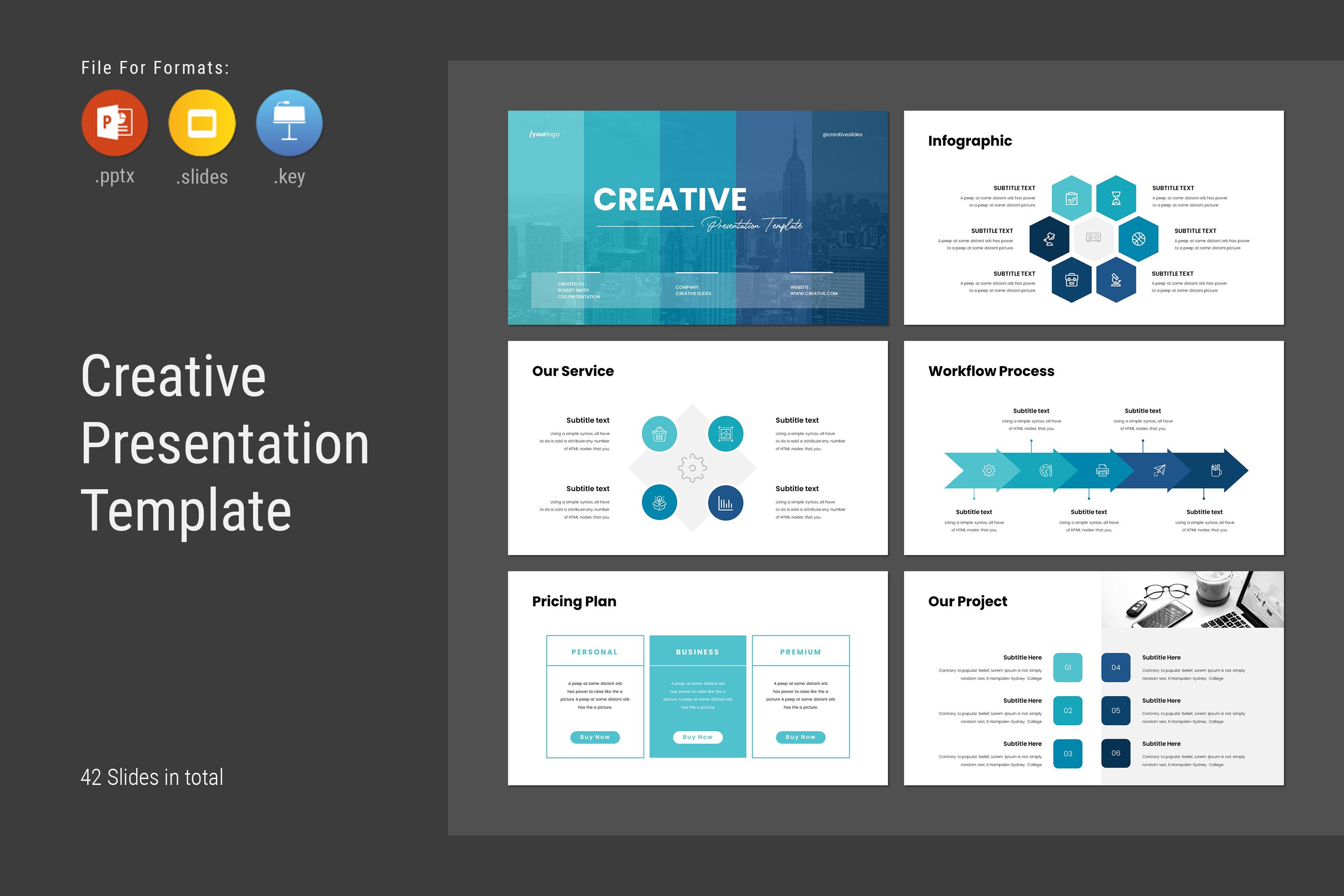The image showcases a Creative Presentation Template designed for PowerPoint, Google Slides, or Apple Keynote formats. On the left side, under a dark gray background, there's a section that lists file formats (PPTX, Slides, Key) with corresponding red, yellow, and blue icons. Below this, white text reads "Creative Presentation Template," followed by "42 slides in total" in smaller print. 

To the right, set against a lighter gray box, is a preview comprising six overlaid slides. The coverslide features a gradient transitioning from aqua blue to dark blue over a New York City skyline backdrop, titled "Creative Presentation Templates." The subsequent slides, each headed with titles like "Creative," "Our Services," "Infographic," "Workflow Processes," "Pricing Plan," and "Our Projects," contain charts, graphs, and detailed content. Slides dive into topics such as service explanations, workflow structures, and pricing plans categorized into personal, business, and premium tiers. The overall theme employs a consistent green and blue color scheme, providing a cohesive visual aesthetic.